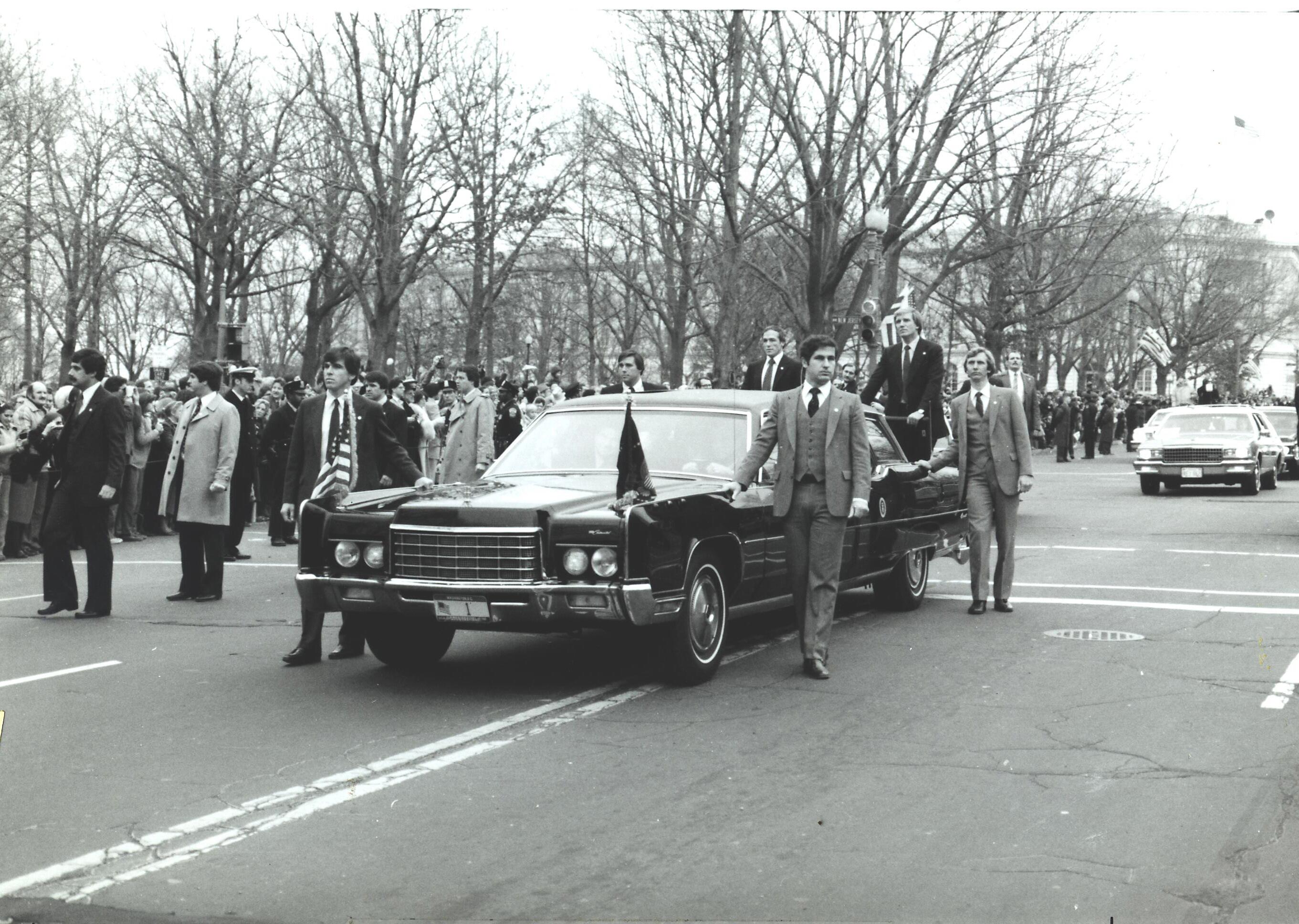This black and white photo appears to depict a mid-20th century parade, possibly from the 1940s to 1960s. The atmosphere suggests a somber or highly significant event, given the formal posture of the individuals and the presence of American flags adorning a central vehicle. The scene unfolds in winter, as evidenced by the leafless trees lining the street. In the foreground, a long, vintage car—potentially transporting a high-ranking government official—commands attention. Several men are positioned around this main car, possibly acting as security personnel, with one individual notably standing on the rear bumper. The car is flanked by other similarly old-fashioned vehicles in the background, reinforcing the period feel of the image. Onlookers crowd the sidewalks, watching the procession, adding to the sense of a communal, public event, potentially a parade celebrating a significant American figure or holiday.